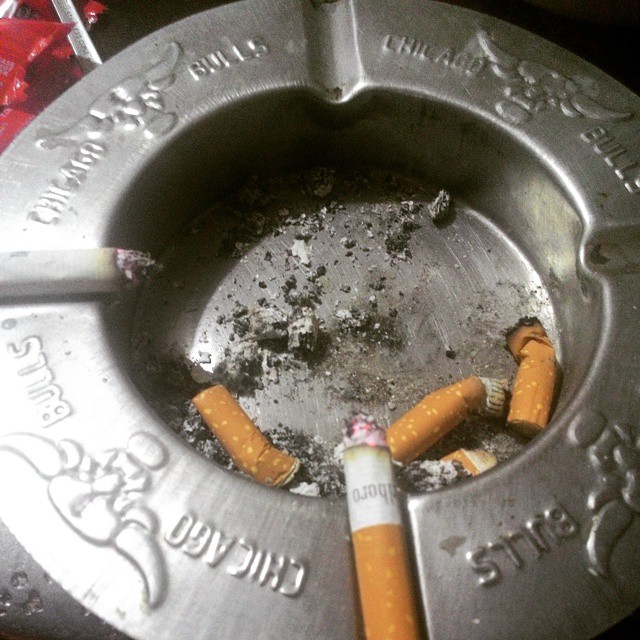This image is a highly detailed, close-up photograph of a round, stainless steel ashtray, featuring etched text and imagery. The ashtray, which has flat, raised edges and a sunken center like a bowl, prominently displays the words "Chicago Bulls" engraved around its circumference, with the team's bull symbol appearing between the text in four sections. The ashtray includes four slots designed to hold cigarettes, and the interior is littered with ashes and four orange-filtered, white cigarettes that have been put out. Additionally, a partially smoked cigarette with the brand name "Marlboro" (partially visible in black font) rests in one of the grooves along the edge, with the faintly lit end suggesting recent use. A bit of red is faintly visible in the upper left background, adding a subtle touch of color to the otherwise monochromatic focus on the ashtray and its contents.